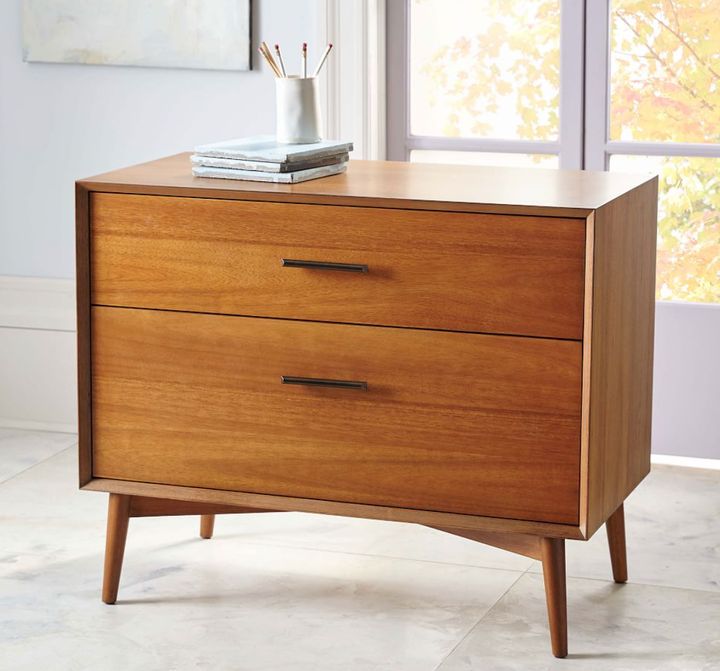The photograph captures a mid-century style wooden desk with two drawers, characterized by its horizontal dark handles and four legs. The desk's wood exhibits a light to medium color, suggestive of 1950s or 60s design. The top drawer appears slightly larger than the bottom one. Positioned on a white marble-tiled floor, the desk sits against a backdrop featuring a pair of off-white walls and a double-pane glass window. Outside the window, out-of-focus trees display vibrant yellow and red leaves signifying autumn.

On the desk's surface, a small white mug holds five pencils—three white and two yellow—while three white DVD cases (or possibly book-like items) are stacked beside it. To the top left of the frame, an abstract blank canvas can be seen, adding a subtle element of art to the scene. The atmosphere hints at a serene, minimally decorated space with a modern vintage touch.